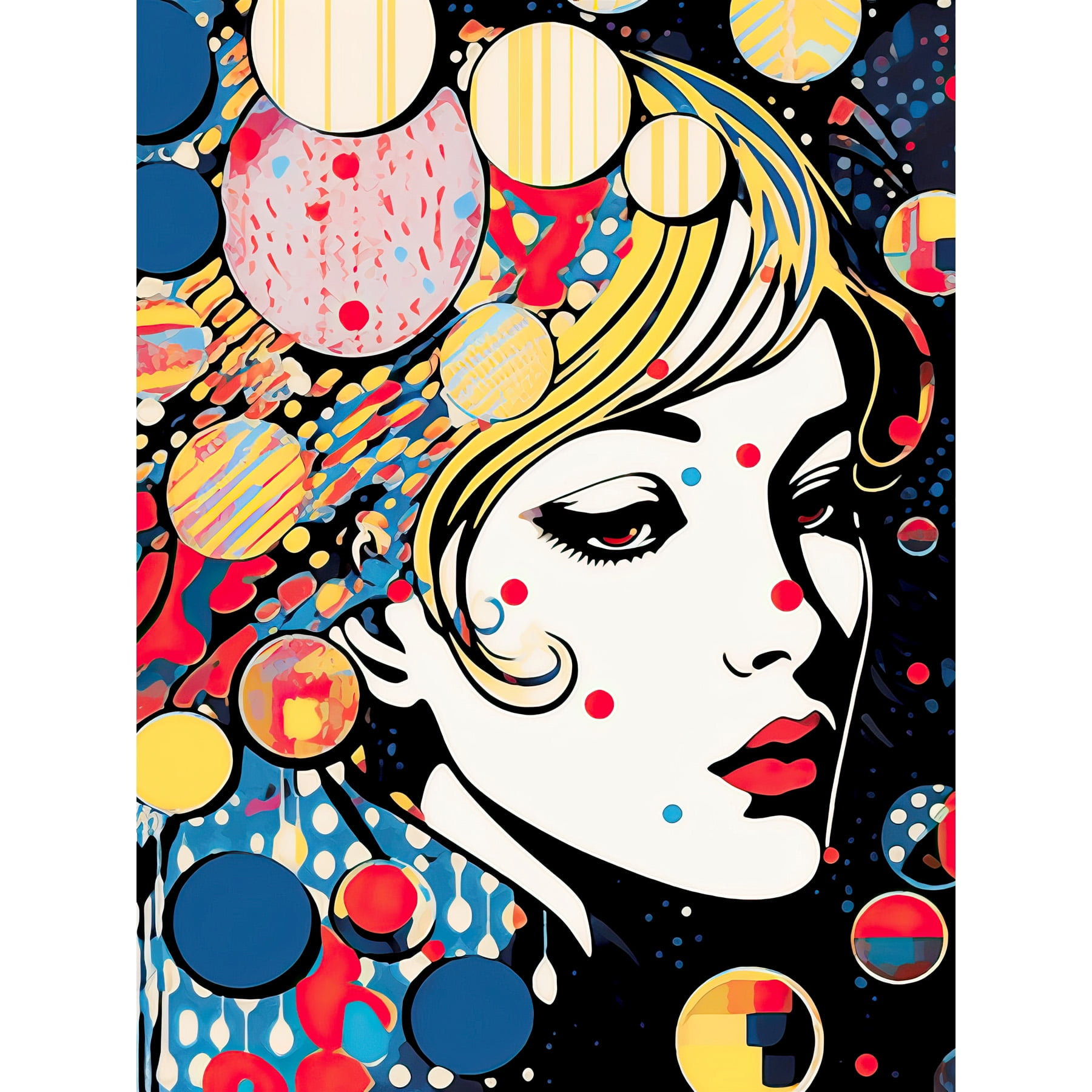The painting is an abstract, pop art-inspired depiction of a woman's face, characterized by its cartoonish, animated style. The piece is vertically rectangular, featuring a predominantly white face with red eyes and bright red lips. Her blonde hair partially curls towards her eyes, adding to the stylized nature of the image. Scattered across her face are red and light blue polka dots, enhancing the whimsical aesthetic.

The background is a vivid tapestry of colors and patterns, dominated by circles and ovals of varying sizes and designs. On the bottom and right parts, a black background showcases yellow designs within the circles, along with blue and red ones. Moving left, the circles become larger, with many being white with yellow vertical stripes. Additional elements include solid blue circles, and a few more with yellow stripes.

Behind the figure's head, the abstract patterns intensify—white backgrounds with yellow stripes, pink ovals with red dots, and a mixture of blue and red dots and stripes. The woman's shirt appears partially in the frame with a white and black collar and a shoulder area that is blue with white polka dots. The front right side of the painting is predominantly black, filled with blue, white, and pink polka dots, adding to the dense, energetic composition of the piece.